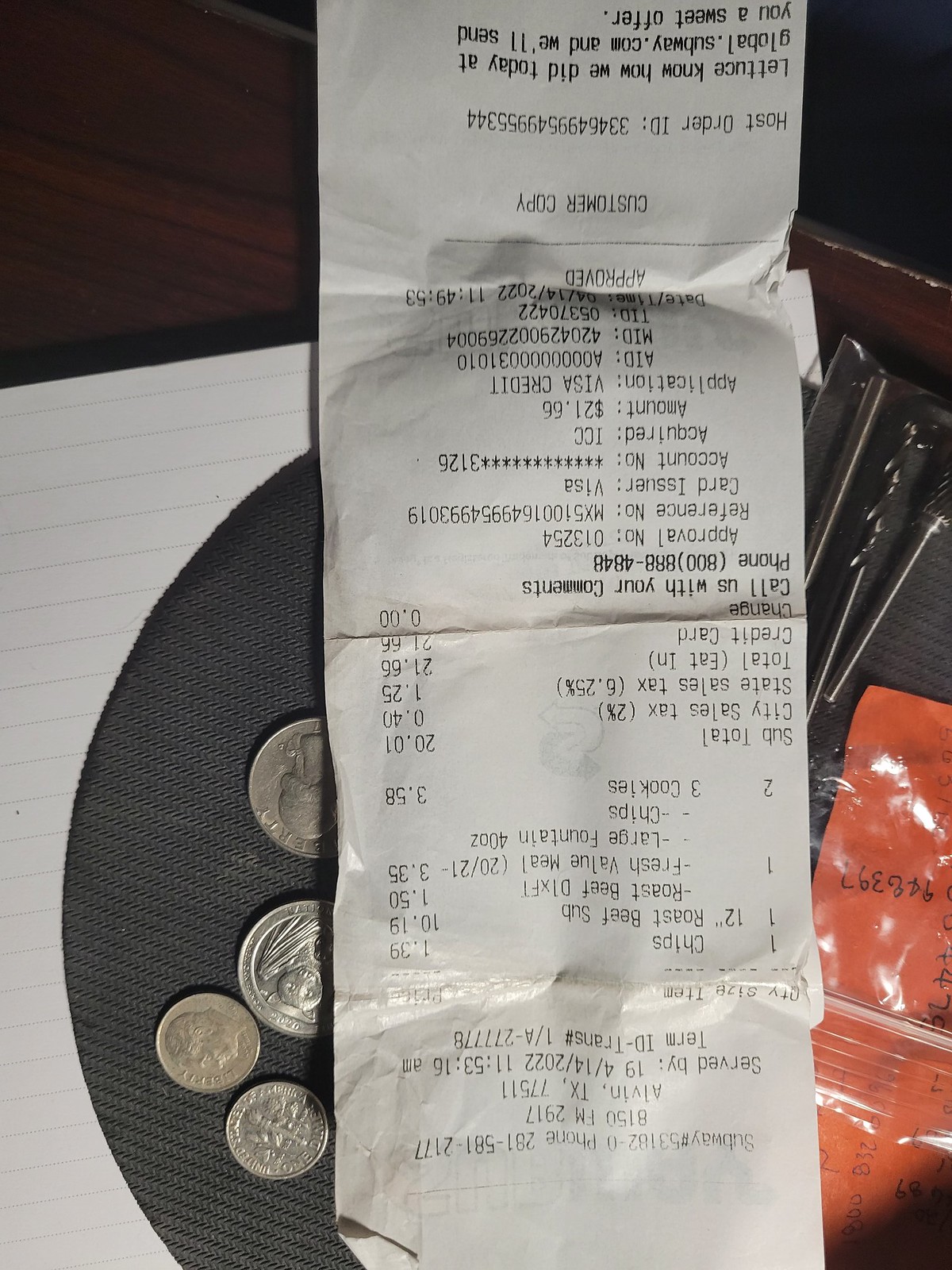The photograph depicts various items scattered atop a dark, reddish-brown wooden table. The centerpiece of the image is an upside-down Subway receipt listing items like chips, a roast beef sub, a fresh value meal, a large fountain drink, 40 ounces of chips, and three cookies, amounting to a subtotal of $20.01, with an added tax of $1.25 for a total of $21.66. The receipt is prominently marked "customer copy" at the bottom.

Beneath and slightly overlapping the receipt are a few coins—two quarters and two dimes—resting on a circular gray fabric placemat. This placemat sits atop a lined sheet of notebook paper, partially obscured. Adjacent to the receipt on the right side, there is a small plastic bag containing black items that resemble drill bits. Accompanying these items is an orange piece of paper with numbers inscribed on it, further adding to the assortment of objects. The upper right corner of the receipt slightly curves off the edge of the table, emphasizing its textured surface.